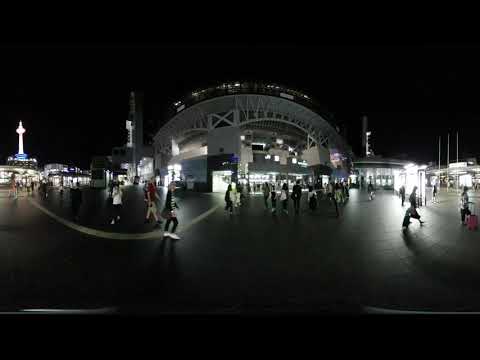The photograph captures a nighttime scene in an outdoor walking area, illuminated by artificial lights that reflect off the shiny, flat ground. A crowd of people, some dragging suitcases and carrying bags or purses, are moving in various directions, suggesting a busy, possibly urban environment. In the foreground, there is a prominent white building with a curved, possibly arched rooftop, giving the impression of a stadium or similar large structure. The image is distorted with a curved effect, possibly due to a filter or a special type of lens. Adding to the complexity of the scene, the photograph includes horizontal black strips at the top and bottom, framing the mysterious and bustling nighttime activity.